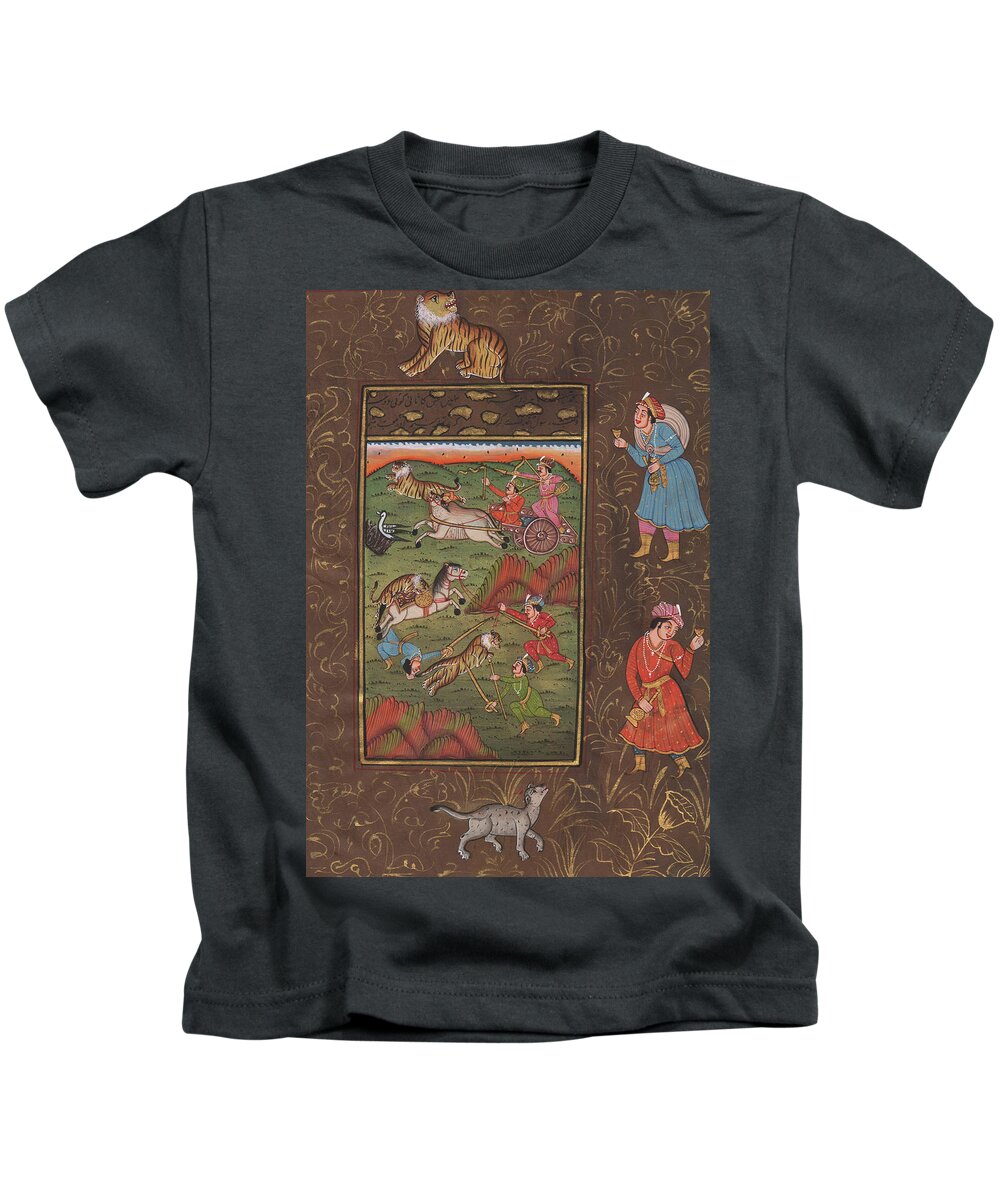This photograph captures a black t-shirt laid out flat, displaying an intricate design that stretches from just beneath the collar to a few inches above the waistband. The central design, rendered in a rich brown with gold floral filigree, frames a complex illustration reminiscent of Persian miniature art. At the top of the rectangular image sits a tiger, establishing a regal tone. Below, a dynamic battle scene unfolds where men in turbans and robes, some on horseback and possibly in chariots, engage in a hunt for lions. This scene suggests an ancient or medieval narrative, possibly involving a king. Additional smaller elements enrich the design: a civet-like cat or grey cat adorns the bottom, and sketches of papyrus are etched in an orangey-yellow hue in the background. Other notable figures include a man hunched over with a pack, a person holding a small glass of wine, and a pair of medieval-looking individuals off to the right, one clad in a red robe and the other possibly a woman in a blue dress. The t-shirt combines these eclectic elements into a scene that melds historical and mythical imagery, creating a piece that is both unique and visually captivating.